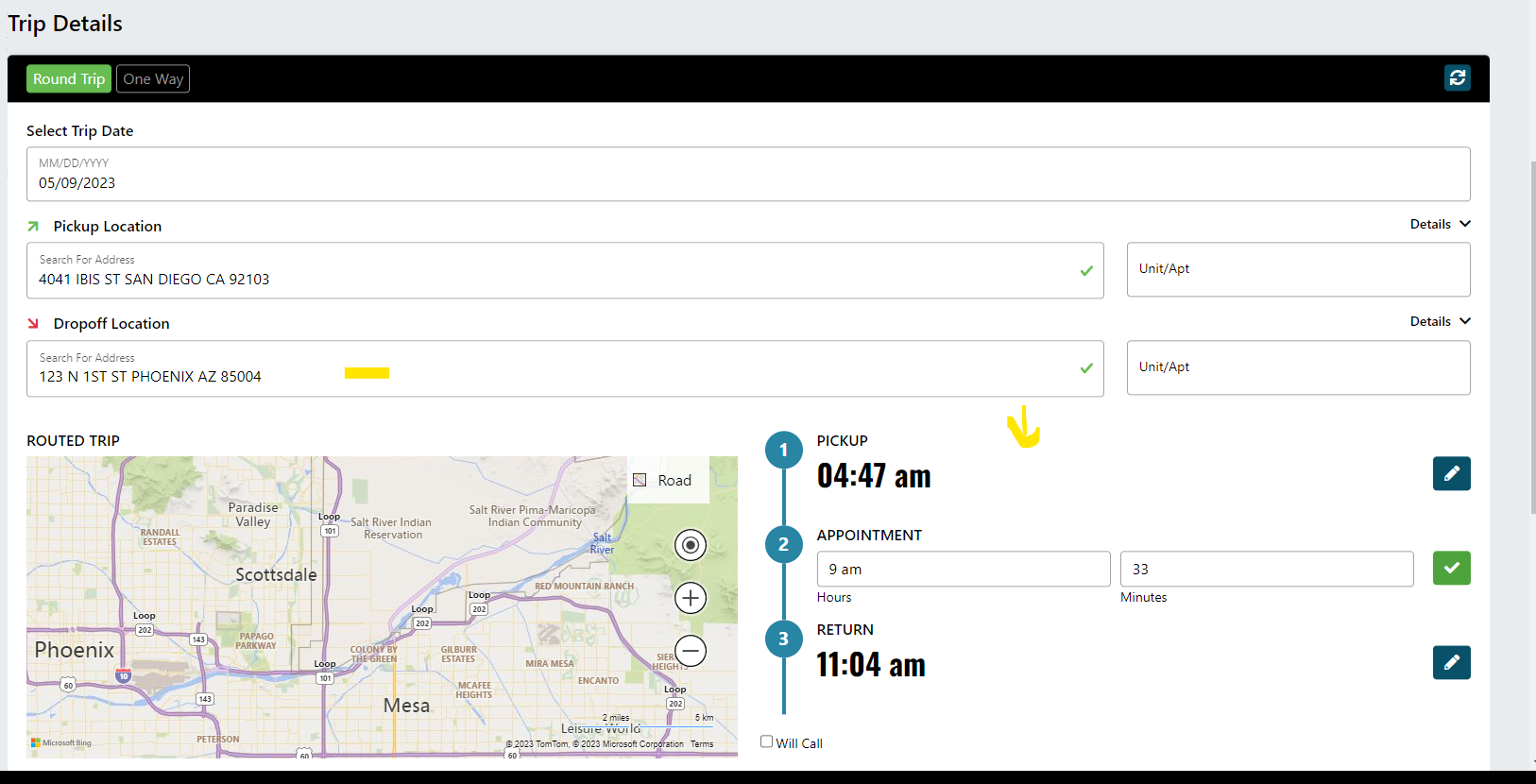The image displays a screenshot of a trip details platform. In the top left corner, the text "Trip Details" is prominently displayed with a capital 'T' and 'D'. Below this heading, a black title bar features three important elements: a green "Round Trip" button on the left, a greyed-out "One Way" button in the middle, indicating it's not selected, and a reload icon on the far right.

Beneath the title bar, user input fields are neatly arranged. The first input field is labeled "Select Trip Date" and it is currently set to "05/09/2023," displayed in the mm/dd/yyyy format. Next, there are fields for trip locations indicated by icons and text. An icon resembling an ascending airplane signifies the "Pickup Location," with the address "444041 Ibis Street, San Diego, California, 92103" entered in the input box. A check mark at the end of the input box confirms the address entry.

Following this, the "Drop Off Location" section has a similar layout, featuring an input box labeled "Search for address" for users to enter the drop-off point. Below the location fields, there is a section titled "Routing Trip" that includes a map outlining the trip route. Accompanied by textual markers, the map highlights key points: "1. Pickup," "2. Appointment," and "3. Return," denoting the sequence of the travel itinerary.